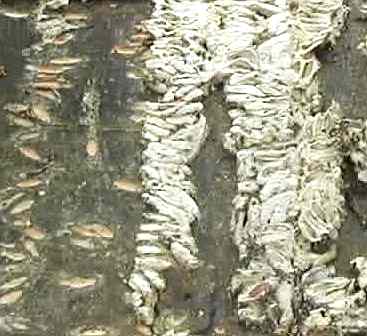The image appears to be a highly blurred and dimly lit color photograph, making it difficult to discern precise details. At first glance, the background presents a grayish-green hue with blurry elements meshed together. On the right side of the image, there are numerous whitish, rectangular, and narrow objects, some of which might be dead fish arranged in piles. These objects are positioned horizontally and appear to connect at the top with additional similar items. On the left, the image becomes slightly more clear, possibly revealing fish still swimming, contributing to a stark contrast between the left and right sides of the photograph. Among these piles of whitish objects, there are also light brown items, adding to the complexity of the scene. The composition somewhat mimics the appearance of tree bark with horizontal lines, valleys, and varying tones of gray, brown, and ivory. The ambiguity of the scene leaves room for it to be misunderstood as a close-up of an unknown substance, perhaps even a section of a painting, with some elements hollowed out and others placed on their side.